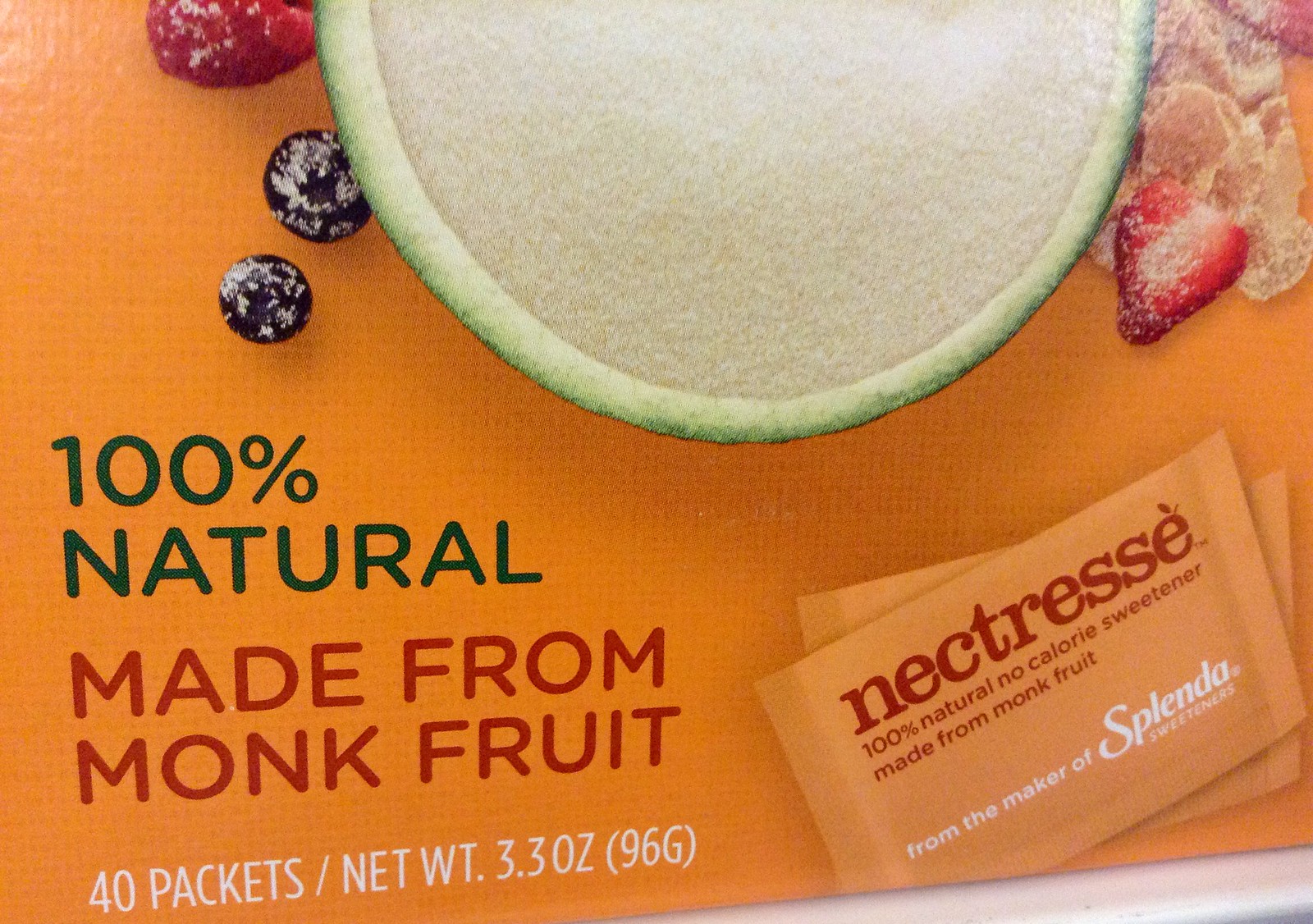**Detailed Captivating Advertisement Caption:**

This advertisement is prominently featured on a piece of paper, zoomed in to showcase a vibrant and inviting scene. At the forefront is a generous, white bowl brimming with sweetener, encircled by a colorful assortment of fresh berries, including strawberries, blueberries, and raspberries. Nestled among the berries are a few pieces of cornflake cereal, adding a touch of breakfast appeal.

Centered at the bottom of the image, the recognizable Splenda logo is prominently displayed in white. Above this, text proudly announces, "From the makers of Splenda Sweeteners."

Dominating the top portion of the advertisement in bold letters is the brand name, "NECTRESSE," spelled out as N-E-C-T-R-E-S-S-E. Accompanying this is the claim, "100% Natural No Calorie Sweetener Made from Monk Fruit," emphasizing its healthy, natural origins.

In the bottom left corner, further details solidify its natural credentials: "100% Natural, Made from Monk Fruit." The package information specifies the quantity: "40 packets / Net Wt. 3.3 ounces (96 g)." 

Overall, the advertisement effectively communicates the product's natural, low-calorie attributes, appealing to health-conscious consumers with its clear and detailed presentation.